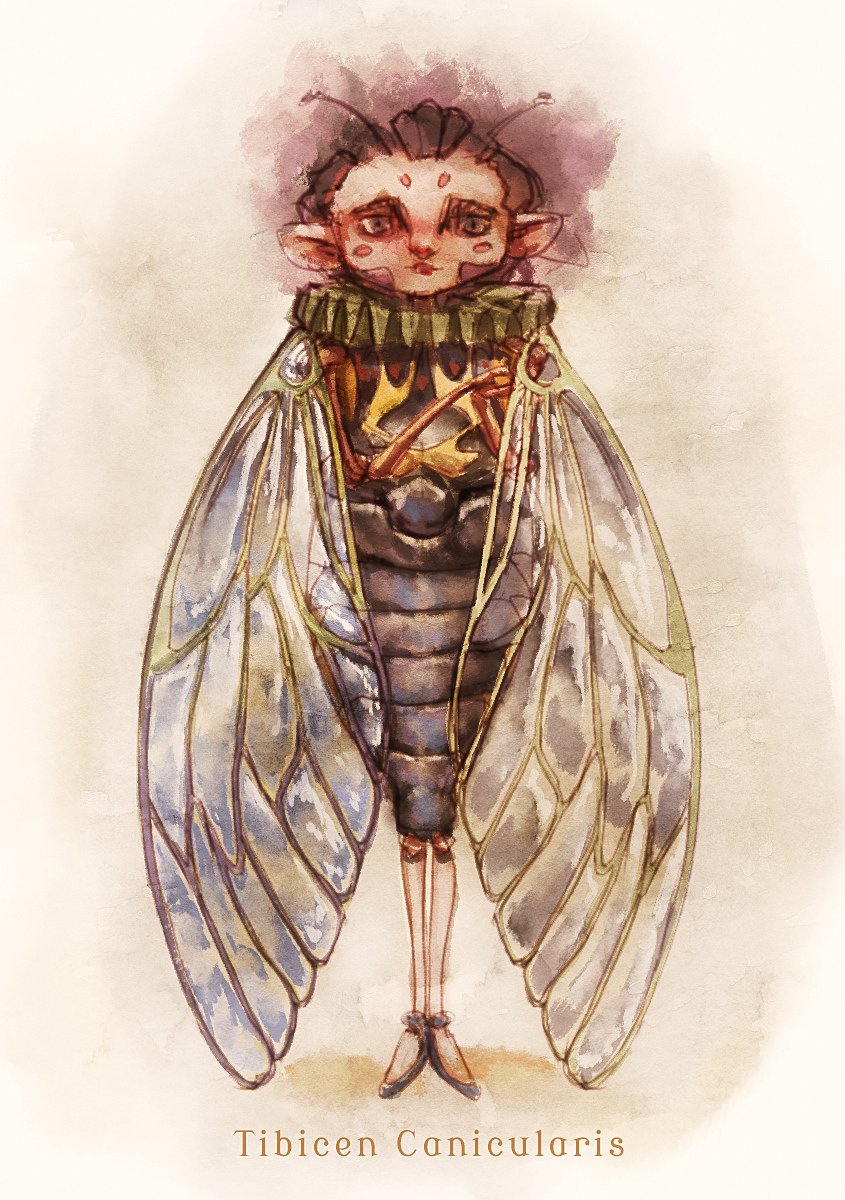This detailed watercolor illustration by an artist creatively combines the form of a human child with the characteristics of a fly. The child retains a human head and legs, which are notably thin and end in pointy shoes, but the rest of the body is distinctly insect-like. The head features a childlike face with slightly pointed, elf-like ears, short wavy brown hair, and two short antennas sprouting from its crown. Around its neck is a green crimped collar similar to what a clown might wear. 

The torso of the figure presents a black, rounded, and scaly texture reminiscent of a cicada or another flying insect, complete with twig-like, clawed arms. From the shoulders extend two large, translucent silvery wings that drape down and nearly touch the ground.

The color palette of the painting is varied, with notable hues of pink, brown, purple, white, and hints of yellow, blending seamlessly into the paper which has no distinct background. At the bottom of the image, the scientific-sounding title "Tibicen Canicularis" (spelled differently in various accounts as "Tibicen" or "Tibicin" and "Canicularis" or "Cana Colaris") is inscribed in light brown lettering. The combination of human and insect elements and the use of watercolor make this piece both whimsical and surreal.